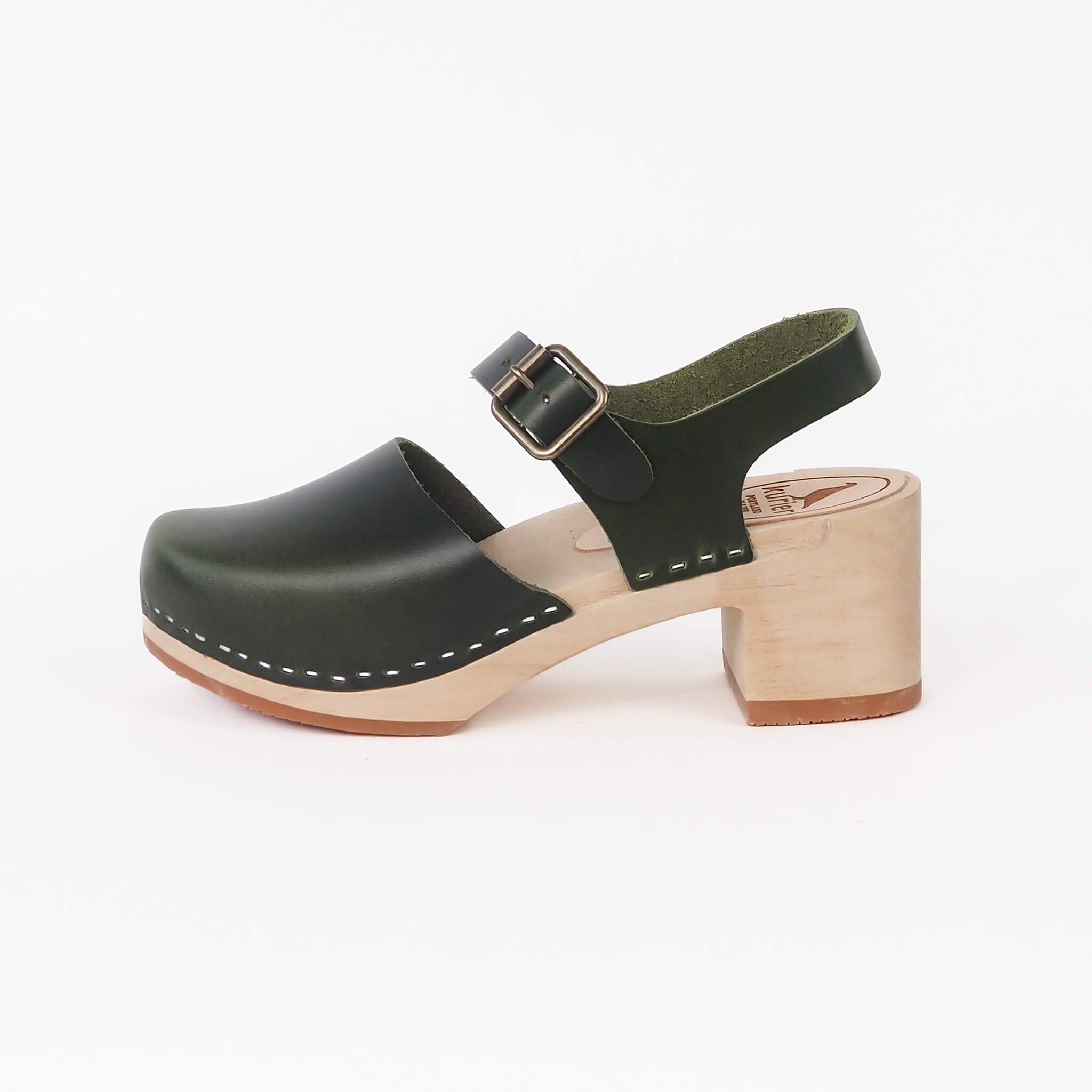This product photograph displays a single women's wooden clog-style shoe against a solid white background. The shoe features a high heel, approximately two and a half inches high. It has a black leather tip and a matching black ankle strap, both adorned with distinct white stitching. The black leather ankle strap wraps over the top of the ankle and secures with a large silver buckle. The shoe’s heel and middle region are exposed, adding to its unique design. The base is crafted from a light brown wood with a dark brown plastic bottom. The brand "Curian" is engraved into the wood near the heel area, accompanied by an intricate silhouette of a bird above the brand name. Additional text is inscribed below the logo, though it is difficult to read. The detailed engraving appears to have been done with precision, possibly through a laser engraving technique.